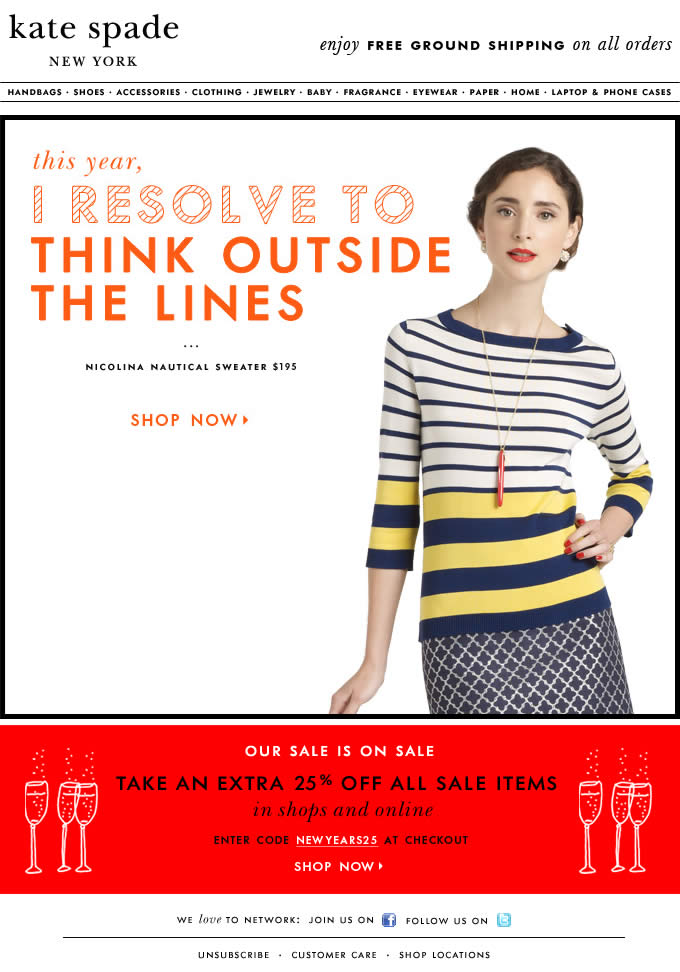This image features a webpage from Kate Spade, New York, set against a predominantly white background. At the top, the Kate Spade, New York logo prominently stands out. To the right, a series of promotional messages are displayed in various fonts: starting with italicized, all-lowercase text, shifting to all-caps in the middle, it reads, "free ground shipping," transitioning to, "enjoy free ground shipping," and reverting back to italicized, all-lowercase with, "on all orders." Below this, a navigation bar offers clickable links (despite being slightly blurred) to categories such as shoes, accessories, clothing, jewelry, baby, fragrance, eyewear, and more.

The central visual highlight is a photograph of a woman styled in a simple, striped dress with three-quarter sleeves, set against a completely white background. Overlaid in bold red text, it features the motivational slogan, "This year I resolve to think outside the lines," accompanied by a "shop now" call-to-action button. 

Directly underneath this image is a vibrant red banner promoting a sale, with white text stating, "our sale is on sale." In black text beneath, it announces, "take an extra 25% off all sale items." Flanking this text are whimsical, hand-drawn illustrations of bubbling champagne glasses, adding a festive touch.

At the bottom of the page, standard footer elements make an appearance, encouraging social engagement with icons for Facebook and presumably Twitter, alongside links to unsubscribe, customer care, and shop locations.